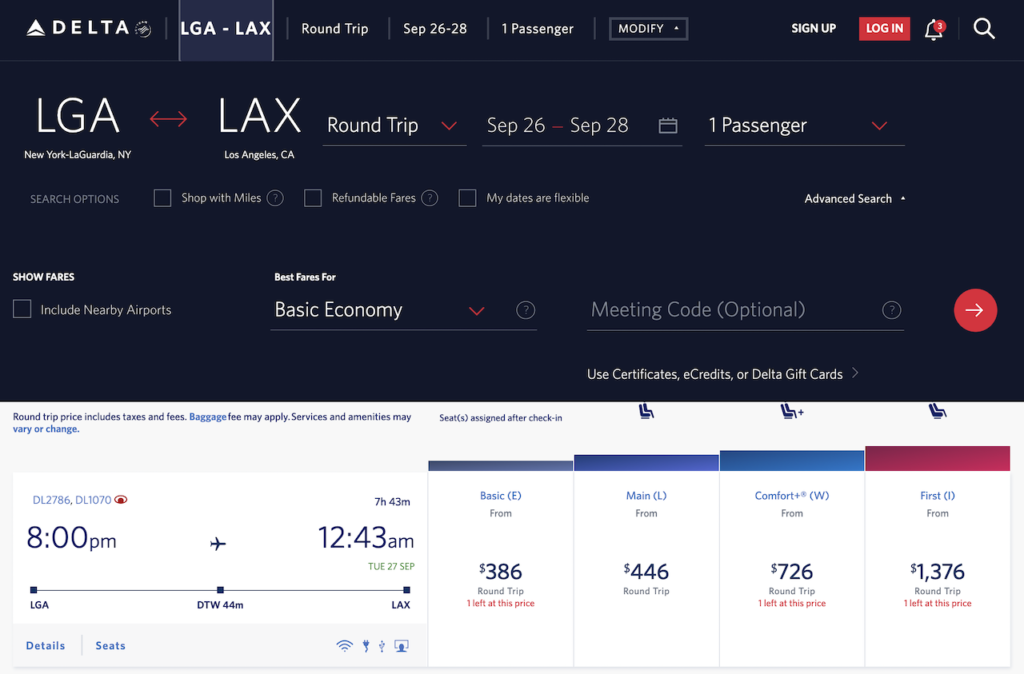Screenshot of a Delta Airlines Booking Page

The screenshot captures a Delta Airlines booking interface. The top two-thirds of the display feature a black background with white text, contrasted by the bottom third, which has an off-white background.

**Top Section:**
- **Top Left Corner:** Delta emblem next to the text "Delta".
- **Flight Info:** Displays "LGA-LAX" indicating the flight route from New York LaGuardia (LGA) to Los Angeles (LAX).
- **Trip Details:** Specifies a round-trip journey scheduled from September 26th to 28th for one passenger.
- **Options:**
  - "Modify" with a drop-down menu.
  - "Sign Up" option.
  - Red "Log In" button with white text.
  - Notification bell icon.
  - Magnifying glass icon for search functionality.

**Middle Section:**
- **Route and Trip Type:** From "LGA" (New York LaGuardia) to "LAX" (Los Angeles, California) for a round-trip (selectable with a drop-down menu).
- **Travel Dates and Passenger Info:** From September 26th to 28th with one passenger (modifiable with a drop-down menu).
- **Additional Search Options:**
  - "Search Options"
  - "Shop with Miles"
  - "Refundable Fares"
  - "My Dates Are Flexible"
  - "Advanced Search"

**Bottom Section:**
- **Fare Options and Preferences:**
  - "Show Fares"
  - "Include Nearby Airports" with a checkbox.
  - "Best Fares for Basic Economy" with a drop-down menu.
  - "Meeting Code" (optional).
  - "Use Certificates, eCredits, or Delta Gift Cards"

**Fare Breakdown:**
- **Time and Class Options:** Displayed fares for different classes: Basic Economy, Main, Comfort, and First Class.

This detailed caption provides a comprehensive overview of the Delta Airlines booking page layout and functionalities.